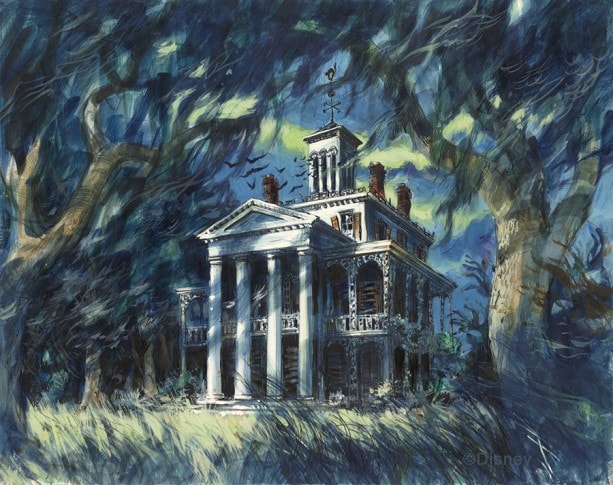This painting depicts an imposing, three-story English colonial-style house with a mixture of Roman architectural elements, contributing to its grandiosity. The house features a prominent white portico supported by four bold columns, creating a two-level porch adorned with intricate white wrought iron railings and arches that frame the bottom two stories. The house exterior is painted white, with windows framed by brown shutters, and is topped with a third floor and a distinguished cupola, complete with four columns and a weather vane.

Three brick chimneys are visible, hinting at a likely fourth hidden behind the cupola. The surrounding scenery suggests an eerie, abandoned atmosphere, with the house enveloped by large, shadowy trees that have fuzzy, blackish leaves. A field of light green grass extends in front of the house, its long blades adding to the neglected feel. The nighttime setting, with a blue-yellowish sky and dark birds flying overhead, amplifies the sinister, almost spooky ambiance of the scene. The overall mood is one of ancient grandeur with a faint touch of haunt.